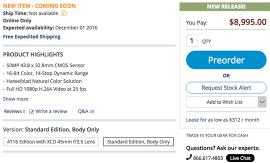The image is a screenshot of an order page, prominently featuring a "New Item Coming Soon" label at the top left. Below this header, there are three lines of text in black. The first line has a circle that appears to contain a question mark. Beneath this, “Free Expedited Shipping” is written in blue text. Following this is a gray bar, under which the phrase "Product Highlights" is displayed.

The "Product Highlights" section contains four lines of hard-to-read text, presumably listing the main features of the product, and is followed by a "Show More" prompt. Below this section, there is black text followed by blue text prompting users to "Write a Review".

To the right, the product details indicate it is the "Standard Edition" and "Body Only" version, along with some serial numbers and other specifics. Adjacent to these details, a "New Release" label in white text set against a green border is visible. Below this, the price is displayed prominently: "You Pay" in black text, followed by " $8,995" in bold red text. The quantity listed is one.

At the bottom, there is a blue button with white text offering options to "Preorder" or "Request Stock Alert", along with an "Add to Wishlist" link. Additional blue text provides further options or instructions to call, signified by a black button.